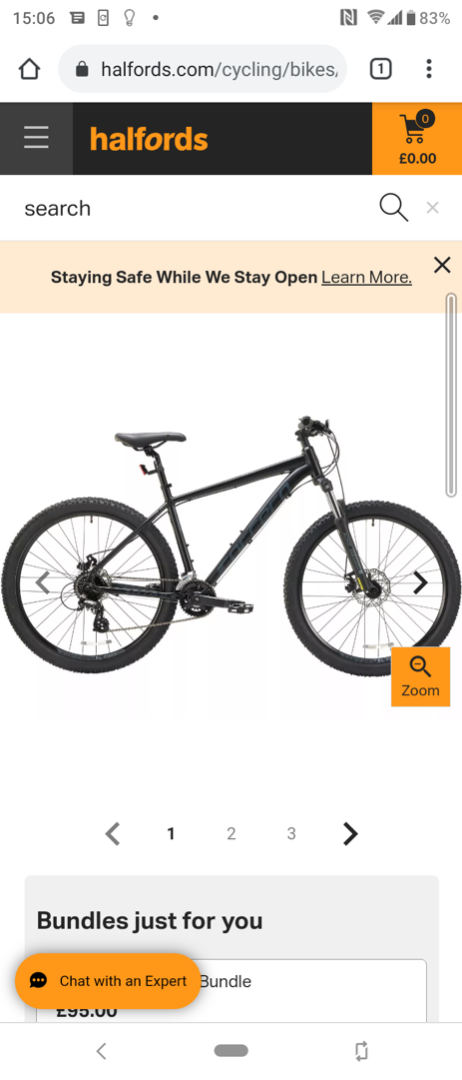An individual is browsing for bicycles on the Halfords website via their mobile device, as displayed at 15:06 military time. The website address, Halfords.com/cycling/bikes, is shown in the address bar. The phone exhibits optimal connectivity and battery status, holding at 83%, and also has one unread message.

The Halfords logo, prominently displayed in orange on a black background, is flanked to the left by a dark grey hamburger menu icon and a black cart icon on an orange background—currently empty. Directly below, a search bar is available for product inquiries. Additionally, a clickable link beneath it reads "Staying safe while we stay open. Learn more," presumably offering information regarding COVID-19 safety measures.

The focal point of the page is an advertisement featuring a sleek, all-black bicycle. The bike has notably large, thick tires, an unusually shaped seat, and straight handlebars. The image is one of three available for viewing, with an option to zoom in for a closer inspection. Below these images, there is a section labeled "Bundles Just For You," which is partially obscured by a button inviting users to chat with an expert for any questions regarding the bike.